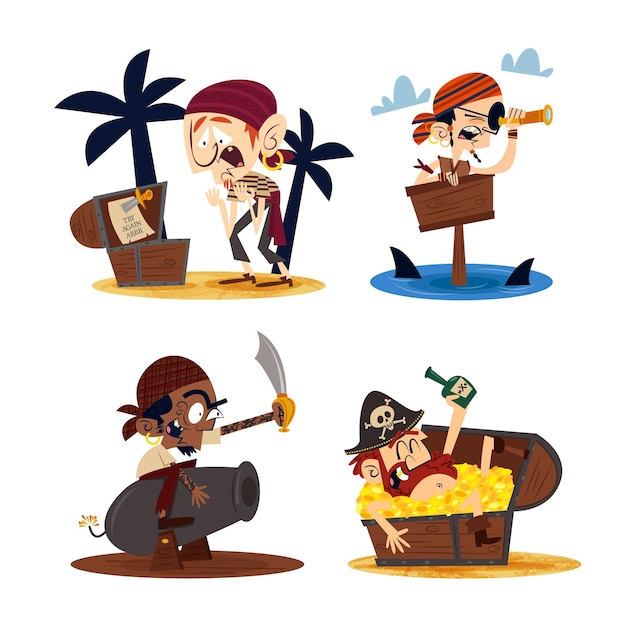This vibrant image is divided into four distinct cartoon illustrations, each featuring a uniquely depicted pirate character. To the left, the first square shows a thin pirate wearing a typical head wrap, screaming with excitement as he stands by a treasure chest amidst two palm trees, likely having just discovered a pot of gold. Next, a pirate balances atop a sailboat mast, surrounded by shark-infested waters. His silly little boat is mostly submerged, with only the mast and shark fins visible, as he keenly scans the horizon through a spyglass. The third scene presents an angry pirate sitting atop a lit cannon, brandishing a knife or sword, ready for combat. This pirate, notable for his dark skin, conveys a sense of intense readiness. Finally, the fourth image showcases a pirate sitting comfortably inside an overflowing trunk of gold. This celebratory pirate, donning a cap, clutches a bottle, probably filled with alcohol, basking in his treasure trove. The illustrations are sharp-edged and vivid, encapsulating a lively and playful pirate-themed adventure.